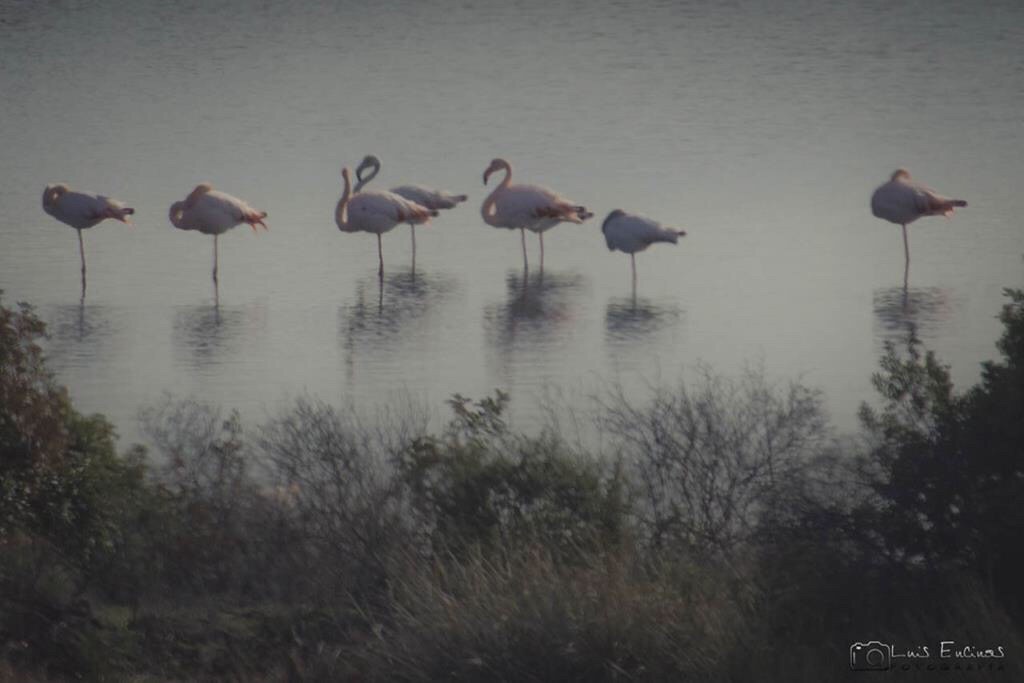This image captures an old, faded photograph of a serene pond surrounded by lush greenery and sparse trees. In the foreground, dense shrubbery frames the scene, with varying patches of green foliage and bare branches. The calm water is home to seven flamingos, standing gracefully, with several balancing on one leg. A few flamingos have their heads tucked under their wings while others have their heads up, visibly displaying their almost grayish-pink plumage, a result of the vintage coloration of the photo. The atmospheric setting appears overcast, contributing to the subdued tones. In the lower right-hand corner, the image is stamped with a camera logo and the name "Luis Encinos," accentuating the nostalgic feel of this rectangular photograph.